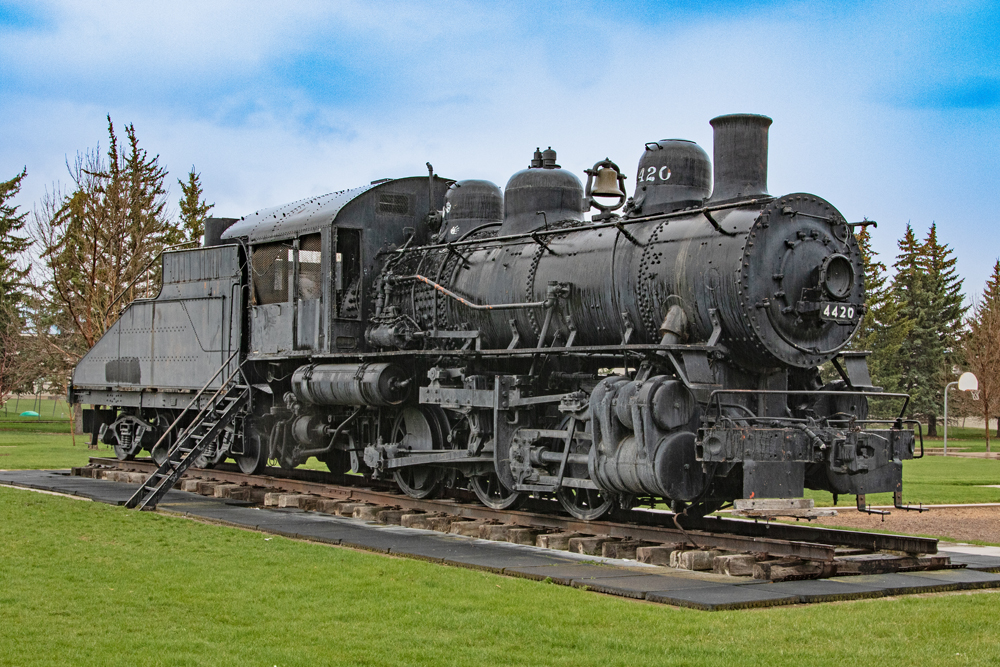This is an image of a black steam locomotive, numbered 4420, situated in a park, likely part of a railroad museum. The train appears weathered, showing spots of rust, and sits on a section of tracks embedded in black rock. Surrounding the train is green grass, and in the background, there are conifer trees under a clear, blue sky. A bell is mounted on top of the locomotive, and there are stairs leading up to the engineer's compartment, suggesting that visitors, especially children, might be allowed to explore it. On the left side of the image, there's a white basketball hoop and a brown bench placed in a playground area with wood chips, adding to the recreational setting of the park.